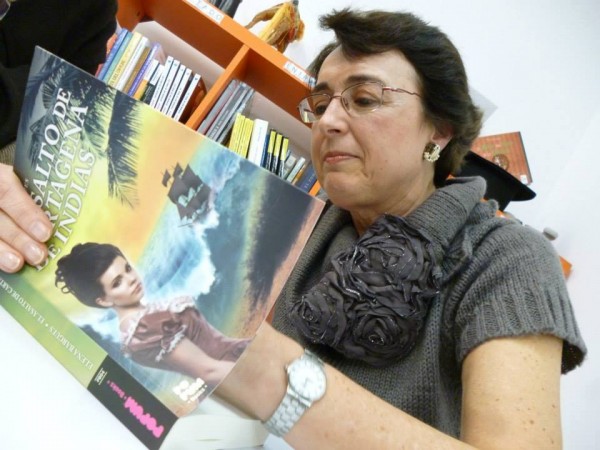The image depicts a middle-aged woman or possibly an author in her 60s, with light skin and short dark brown hair. She is adorned with diamond earrings that feature black and white stones, and she wears glasses with rose gold frames. Her outfit consists of a gray, short-sleeved sweater decorated with a fabric rose pattern around the neck. On her left wrist, she has a silver watch with a white face. She is holding a book, potentially signing it, as another person beside her, wearing a black top, helps keep the book open. The book's cover shows a woman in a burgundy dress by a beach with a pirate ship in the background, hinting it might be a romance or adventure novel. The setting appears to be a library, with bookshelves and a white wall visible in the background.